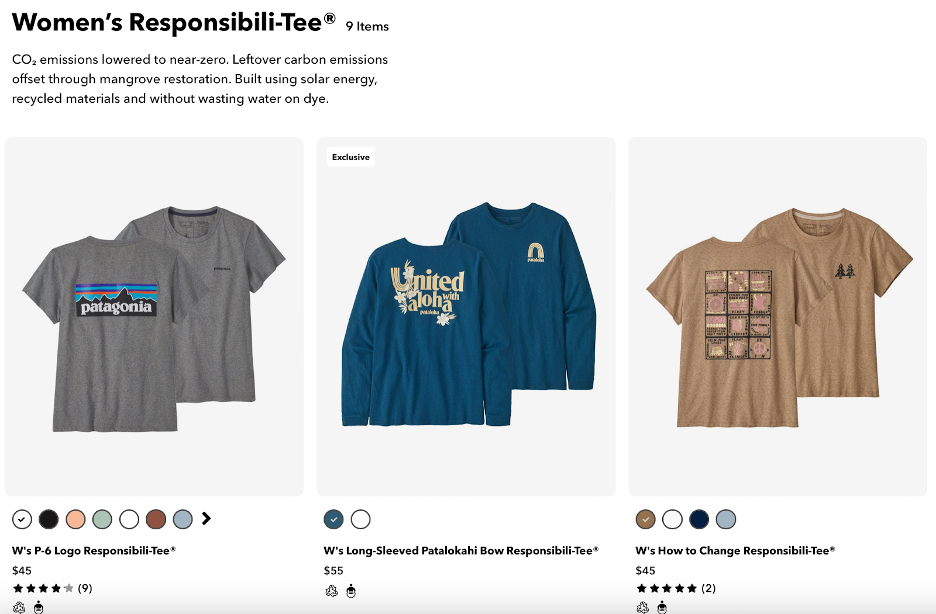This image showcases a section of a website featuring the trademarked brand "Women's Responsibility Tee." On the right, there are details about nine different T-shirts. The website highlights its commitment to sustainability, noting that CO2 emissions are nearly eliminated, with residual emissions offset through mangrove restoration. It further emphasizes the use of solar energy, recycled materials, and waterless dyeing processes in production.

Displayed are three images of T-shirts. On the left is a Patagonia short-sleeve T-shirt in gray. The middle image presents an "exclusive" United Aloha long-sleeve T-shirt in a light green shade. On the right, there are two short-sleeve T-shirts in a light brown color.

Beneath these images are color swatches indicating available colors for each T-shirt. The Patagonia T-shirt is available in black, peach, light green, white, brown, and gray, with a caption stating "W's P-6 Logo Responsibility" priced at $45, boasting a 4 out of 5 stars rating from nine reviews. The United Aloha T-shirt is available only in white or green, priced at $55. The brown T-shirts, priced at $45, are available in brown, white, black, and gray, and have garnered a perfect 5 out of 5 stars rating from two reviews.